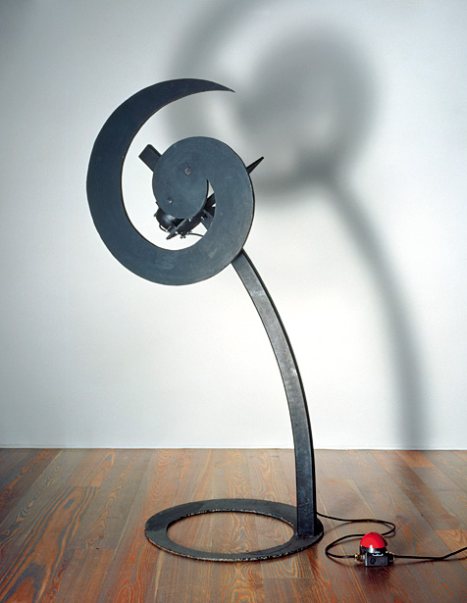The image depicts a black metal sculpture set on a dark brown paneled wood floor, accompanied by a clean white wall in the background that captures the shadow of the sculpture. The sculpture rests on a circular base with a distinctive central cut-out and features a curving pole extending from the right side of the base and bending slightly to the left at the top. At the end of this pole, there's a teardrop-shaped, swirl-like object. Adjacent to this component is a black motor designed to spin the teardrop shape. A black wire runs from the base of the sculpture to a black box positioned at the bottom right, which is fitted with a conspicuous large, red, cone-shaped button. The lighting in the image emphasizes the intricate design of the sculpture by casting its detailed shadow onto the white wall, adding depth and dimensionality to the overall composition.